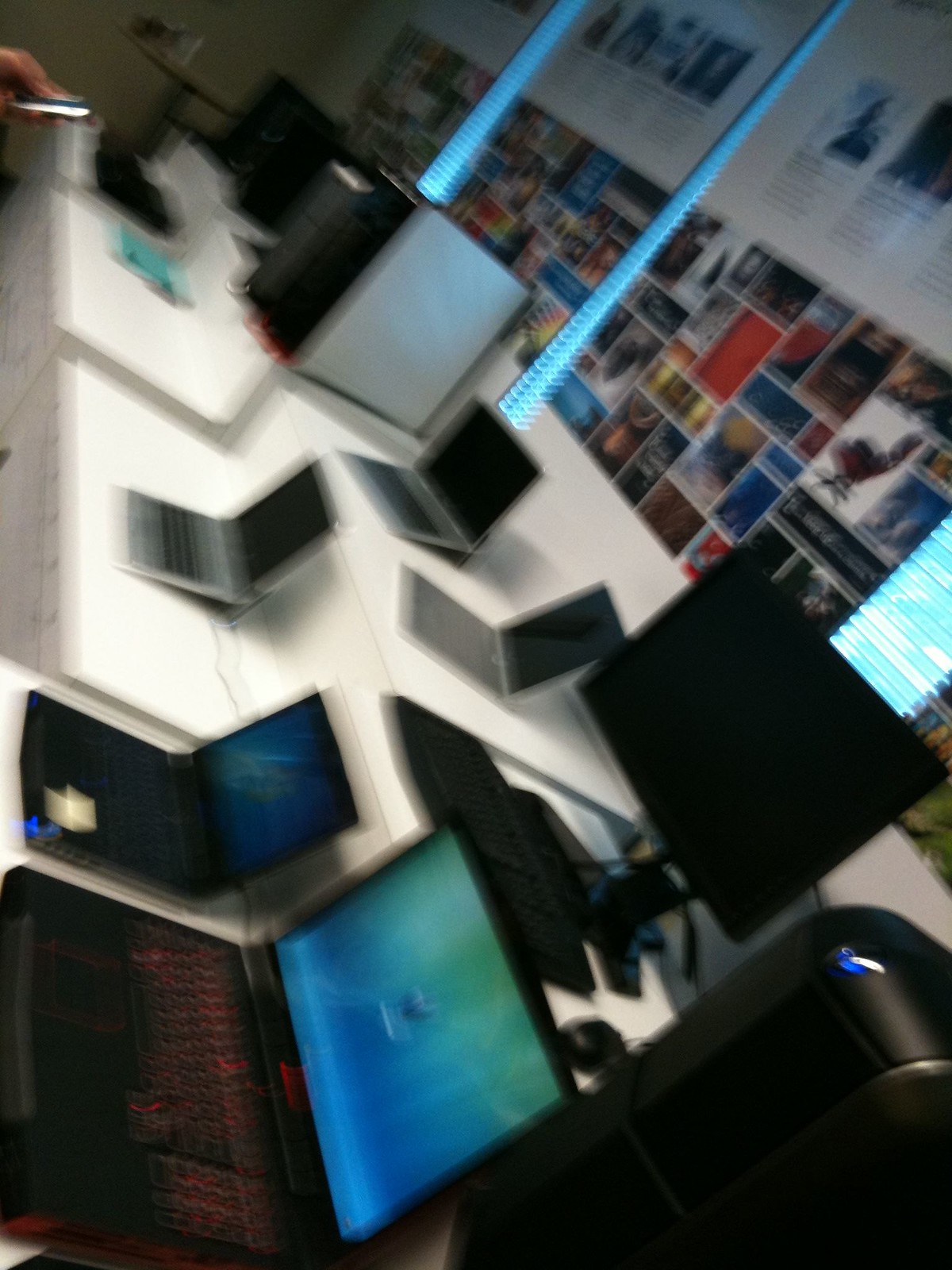The image depicts a blurry, vertically-rotated photograph, suggesting a computer lab or a technical store display. It features at least five open laptops and two desktop computers with monitors, all situated on white, two-tiered tabletops. The scene is cluttered with various black and gray devices, some of which have their screens turned on, displaying blue images suggestive of the Windows interface. The back wall reveals an array of rectangular pictures or posters, interspaced with bright blue LED lights. Additionally, a hand holding a cellphone is visible in the top left corner, pointing towards one of the smaller laptops. The overall blurriness of the image, likely due to camera shake or poor focus, makes fine details difficult to discern.